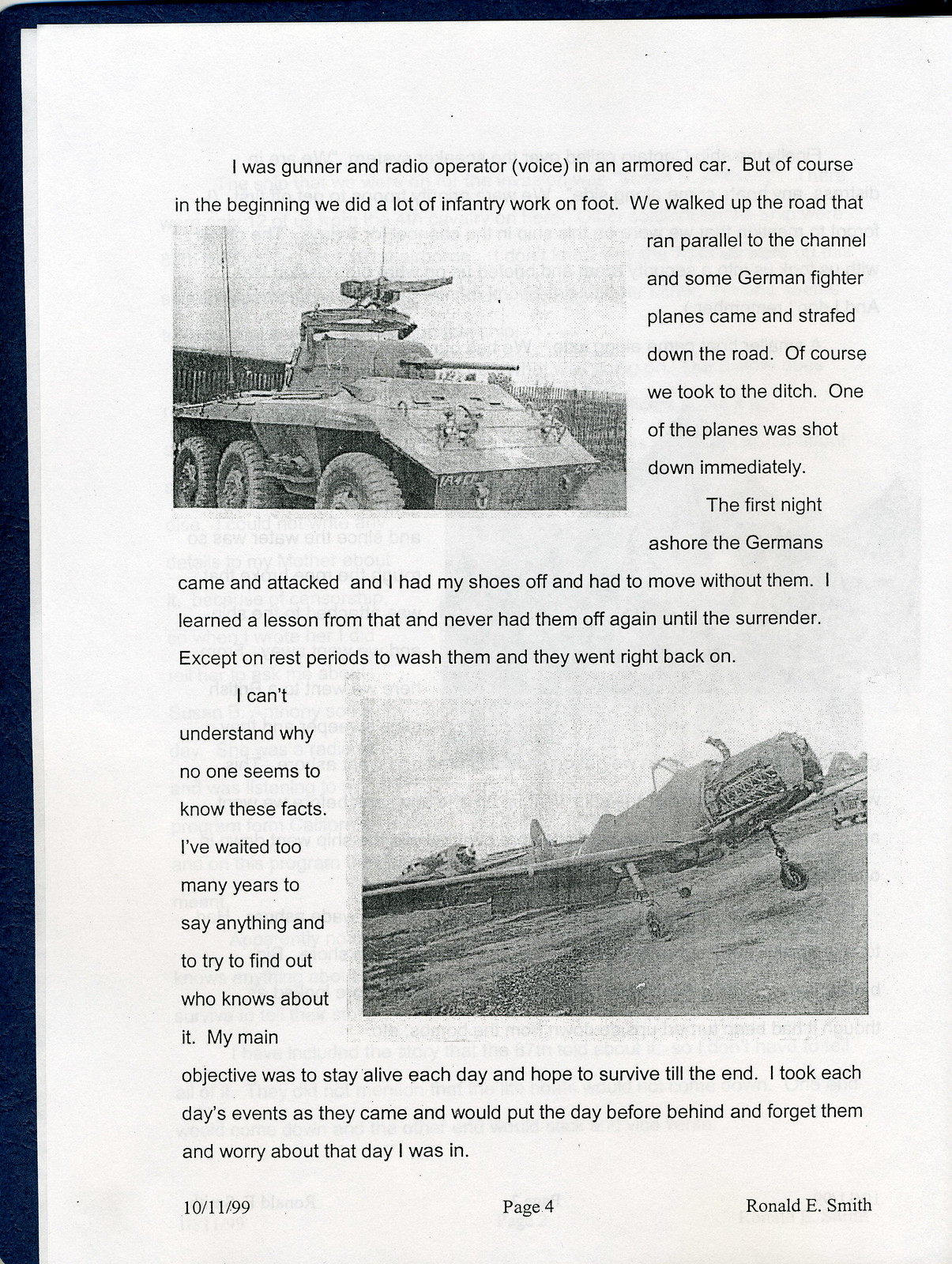This image is a scan of page 4 from a book dated October 11, 1999, authored by Ronald E. Smith. The page is held within a blue binder, visible on the left and top edges. The page features two black and white photographs: the top half showcases an armored car with a turret-mounted cannon and machine gun, adorned with a white star, and text wrapped to the right; the bottom half displays a damaged World War II-era propeller-driven fighter plane with text wrapped to the left. The narrative, presumably a memoir by Ronald E. Smith, recounts his experiences as a gunner and radio operator in an armored car during World War II. He describes initially performing infantry work on foot, moving along roads parallel to the channel, dodging strafing German fighter planes, and surviving a nocturnal attack without shoes. He reflects on the hardship, focusing on his objective to survive each day, documenting his strategy to forget past events and concentrate on the immediate present. At the bottom of the page, the date "10-11-99" is on the left, the page number "4" is centered, and "Ronald E. Smith" is on the right. The overall content seems to encapsulate vivid wartime memories and personal revelations.